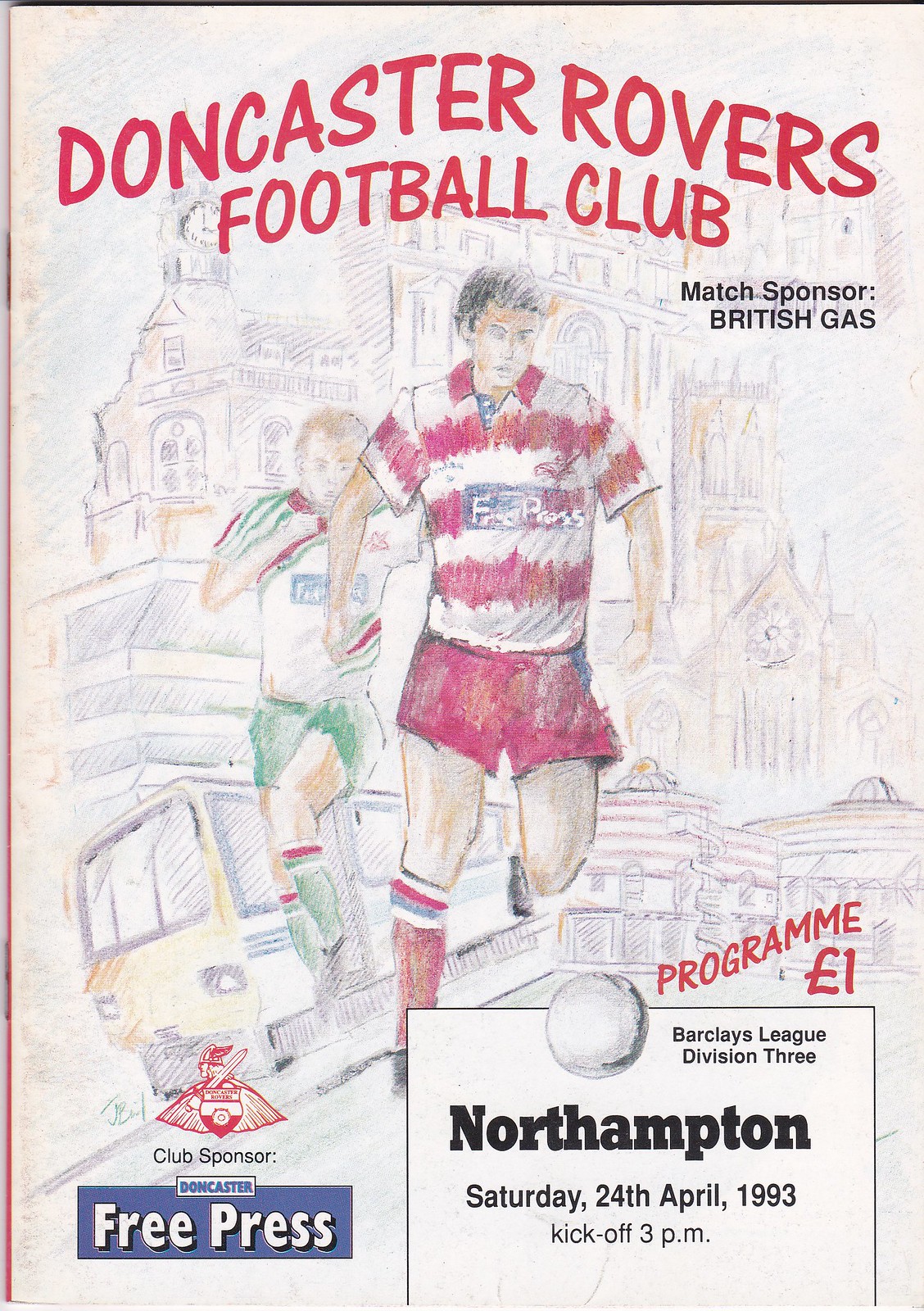The image is a vintage paper program for the Doncaster Rovers Football Club, prominently featuring "Doncaster Rovers Football Club" in red Comic Sans-like font. Below, it states the match sponsor is British Gas and the club sponsor is Doncaster Free Press. The main illustration, rendered in a colored pencil sketch style, depicts a dynamic scene of two football players in action. The foreground player wears a red and white striped kit with red shorts and red socks, chasing after a ball. A trailing player is dressed in a green and white striped kit with matching green shorts and socks. They appear to be playing in front of a backdrop of notable city landmarks, including a large stadium, buildings, and a train. Additional text in the lower right corner announces the match details: "Northampton, Saturday, 24th April 1993, kickoff at 3 p.m.," with "program £1" and the event being part of the Barclays League Division 3.